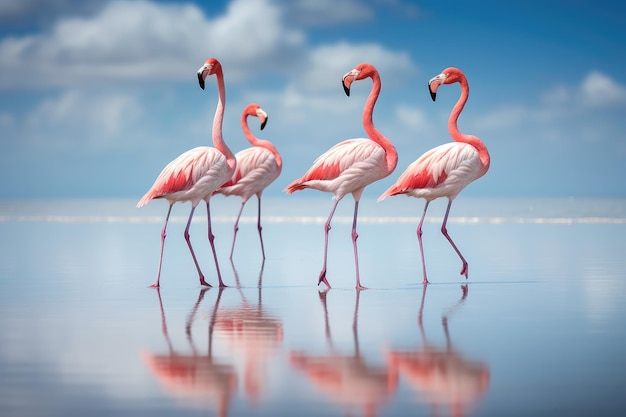In the image, four flamingos are walking gracefully along a wet shoreline, their reflections shimmering in the shallow water beneath them. Each flamingo has long, delicate pink legs and sleek bodies predominantly covered in white feathers, accented with pink wings and red feathers near the edges. Their elegant necks are a striking pink, deepening in color as they reach their heads, which feature long black beaks. The flamingos are positioned with subtle differences— three of them have their heads turned dramatically back over their bodies, while the smallest one looks straight ahead. The background is blurry but it hints at a shoreline meeting the water, with a vivid blue sky dotted by large, puffy clouds above, creating a serene and picturesque setting.